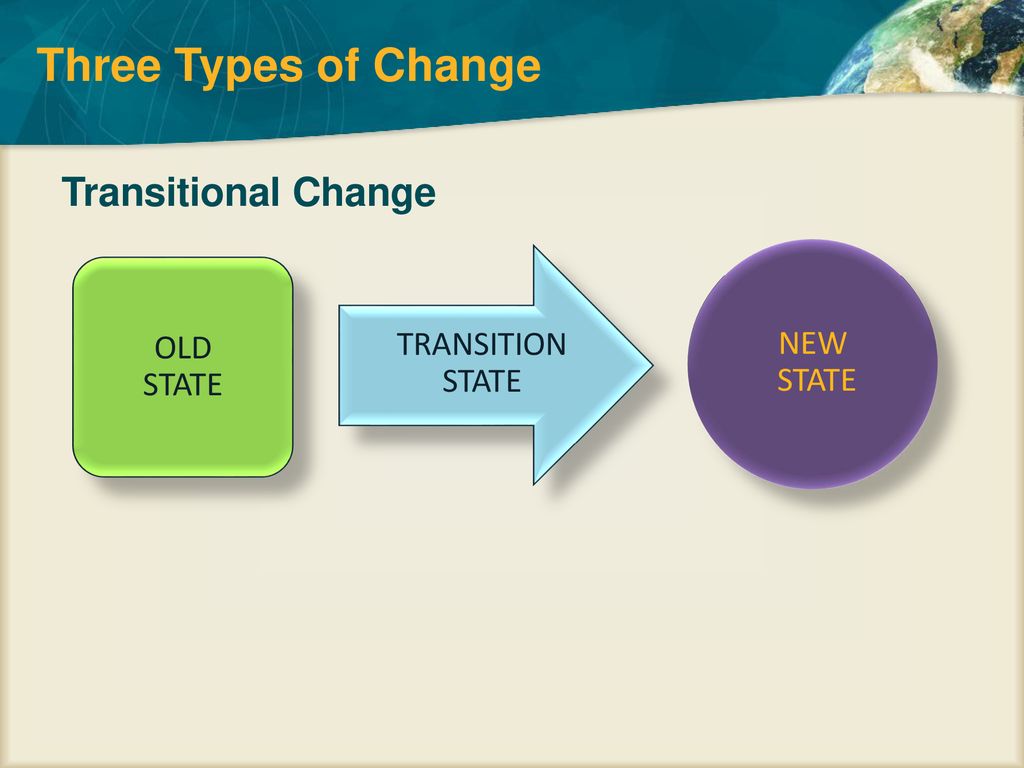The image depicts a detailed flowchart set against a light cream background, illustrating "Three Types of Change" in gold-yellow text at the top, with a dark teal backdrop. Positioned in the upper right is a partial view of Earth, showing the United States and Canada in green and blue tones. Below the title, the flowchart progresses from a light green rounded square labeled "Old State" in dark gray text, through a transitional light blue arrow labeled "Transition State," culminating in a purple circle labeled "New State" in yellow text. The colors used include teal, off-yellow, green, blue, purple, and gray, arranged to create a visually balanced and well-spaced graphic, resembling a slide from a PowerPoint presentation.